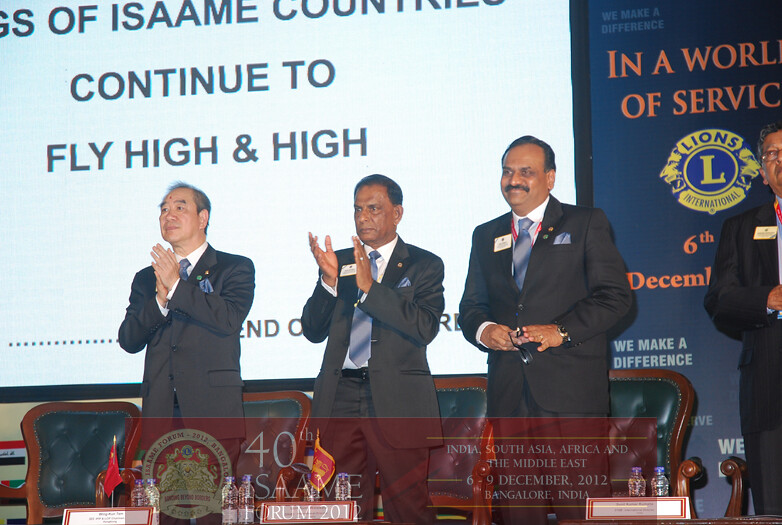In this horizontal rectangular photograph, four men in suits stand on a stage against a backdrop featuring both a large billboard and a projection screen. The men, each wearing dark suits paired with blue striped ties, have name tags on their upper left chests. The man in the middle has his suit jacket unbuttoned. Positioned in front of wooden chairs with green cushions, the two men on the left are seen clapping, while the third man appears to be holding a pair of glasses and the fourth man's hands are out of view. 

The billboard to the right features a dark blue area with red writing that states, "In a world of service," accompanied by the Lions Club logo and some dates. Adjacent to it, on a white section, the text reads, "continue to fly high and high." Superimposed across the bottom of the image, a watermark indicates the event: "40th Isami Forum in Bangladesh, India, South Asia, Africa, and the Middle East, 6th to 9th December 2012, Bangalore, India." Small white and red placards, presumably with the men's names, are placed in front of their chairs. The image overall captures a formal event hosted by the Lions Club International, attended by dignitaries possibly of Asian descent.